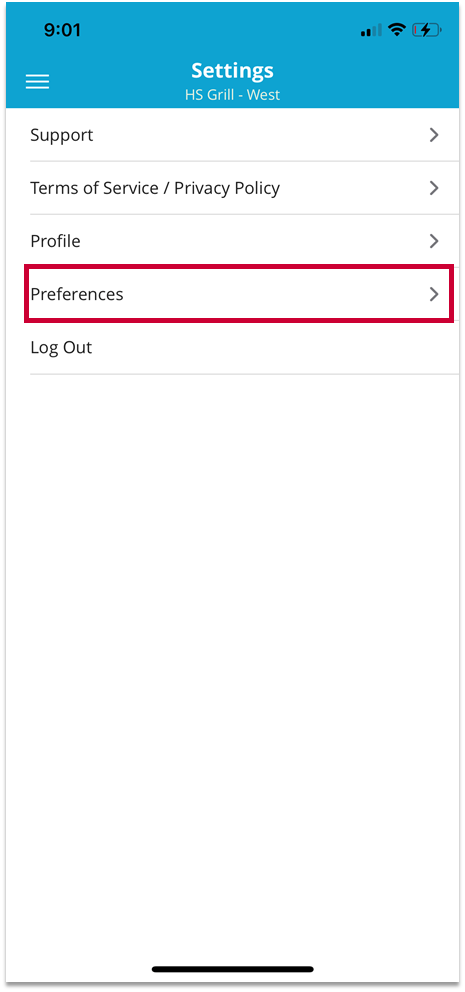This detailed image shows a smartphone screenshot focused on the settings menu. At the very top, the screen has a light blue header occupying the upper two inches. The top left corner displays the current time as '9:01 AM' in black text. To the right, a minimal battery icon with just a thin black line indicates a low charge, though it's being replenished as shown by the charging symbol. The Wi-Fi signal icon is full, while the mobile network signal icon is half full.

Beneath the header is a set of three horizontal white lines stacked vertically on the left side, which typically signifies a hamburger menu. Centrally located in bold white text is the word 'Settings,' followed by the subtext 'HS GRILL-WEST' in all caps.

Entering the main white section, the first item on the list is 'Support,' written in black on the left, with a greater-than sign (>) on the right, demarcated by a thin gray line underneath. The second item is a combined 'Terms of Service / Privacy Policy' also with a greater-than sign on the right, followed by another thin gray line. The third item in the list is 'Profile,' again in black with a greater-than sign on the right, and beneath it is another dividing line.

Further down, there's a prominent red-outlined rectangle labeled 'Preferences' in black text with a greater-than sign to the right. Just below this, a line separates it from the 'Log Out' option, also in black and similarly separated by a thin line underneath.

The entire settings interface has a thin gray border encompassing it. Near the bottom-center of the screen, there's a central gray bar flanked by thin borders, positioned approximately an inch left and right from the center.

This meticulous description captures each element within the screenshot, clearly defining the layout and interactional components of the smartphone’s settings menu.